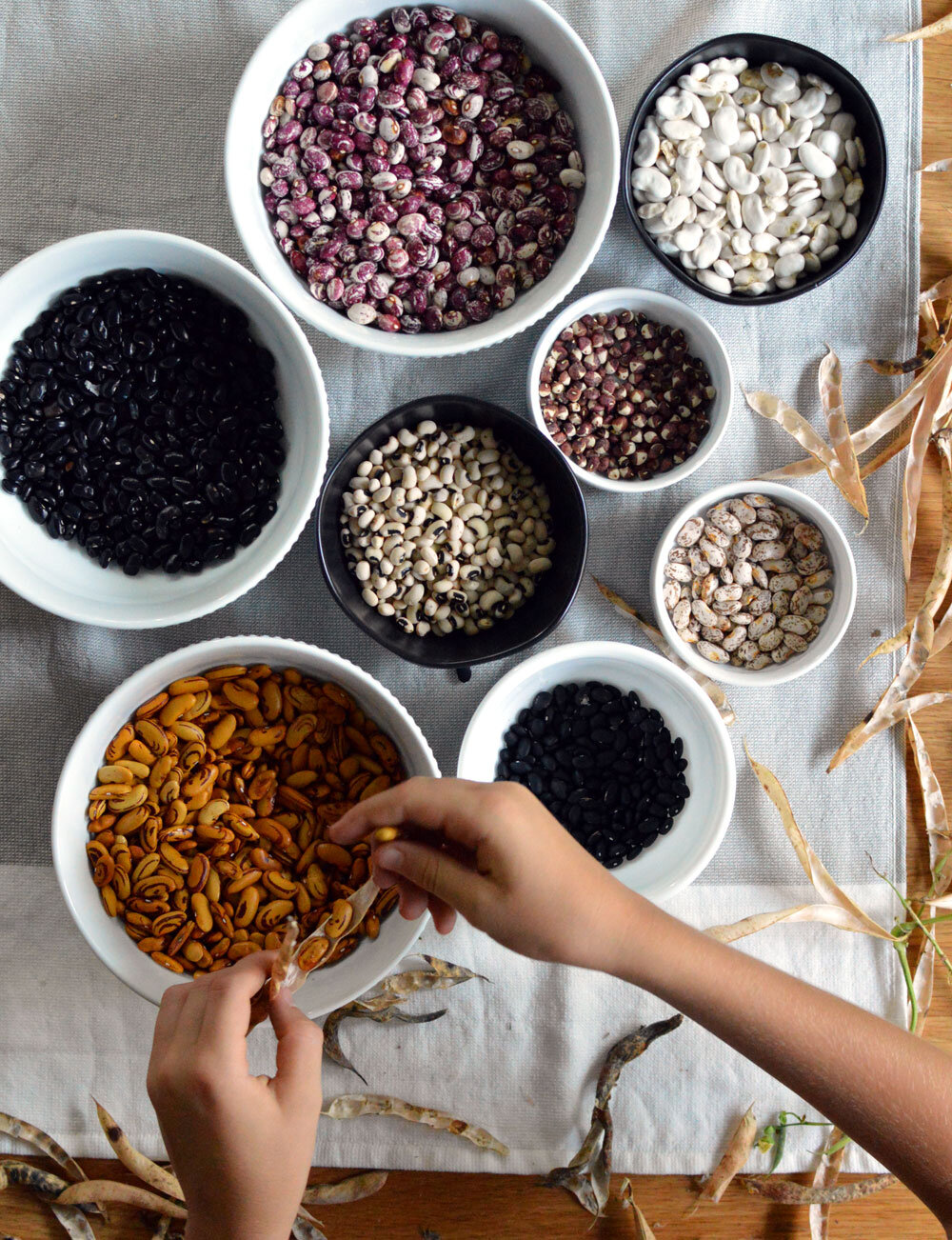This overhead color photograph, presented in portrait orientation, showcases a meticulously arranged flat lay of diverse beans and legumes in various round bowls on a table. The table is partially covered with a white cotton runner and is made of wood. The bowls, differing in sizes from small to large, are primarily white, complemented by a few black bowls. 

Starting from the lower section of the image, two lighter-skinned hands (possibly female, Caucasian or Asian) reach towards a white bowl filled with brown beans, one hand entering from the bottom and the other from the right, appearing to open a seed pod and emptying the brown oval seeds into the bowl. To the right of this bowl, there is a smaller bowl with black beans. 

Moving to the middle of the image, a central bowl holds black-eyed peas. Adjacent to it on the right is a small bowl with black beans, and further up to the right is a bowl of pinto beans. Above these, closer to the center top right, a black bowl contains kidney-shaped white beans. In the upper left section is a bowl of mixed grayish and white colored beans, while the large bowl in the top center holds a mix of brown and white beans. Additionally, the upper left corner features a large bowl filled with black beans.

The arrangement of the bowls on the white linen cloth, adorned with scattered bean pods around its edges, creates a visually appealing representation of various legumes through the lens of food and product photography. The photo embodies elements of representationalism and realism, highlighting the distinct textures and colors of the beans.